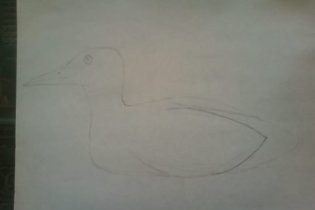A small, horizontal, rectangular image features a delicate pencil sketch of a duck depicted in profile, facing left, on a pristine white piece of paper. The duck is outlined with careful, light strokes, except for intricate details in the eye and beak, which are more defined. The sketch captures the duck from the lower body and wings upward, suggesting it is swimming or floating in a water environment, as no feet are visible. The white paper rests on a dark brown tabletop, a small rectangular section of which is visible, providing a contrast to the simplicity of the drawing.